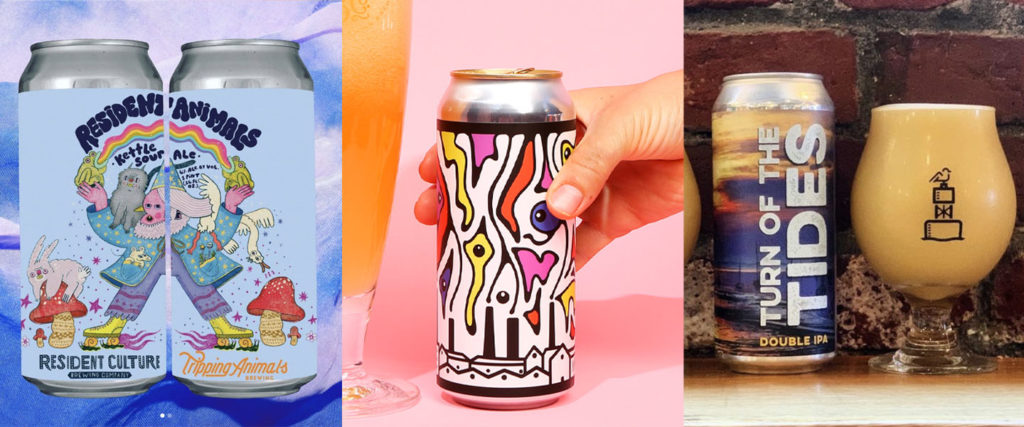The image is divided into three distinct rectangular panels, each featuring cans of beverages. In the first panel on the left, there are two cans side by side that together form the phrase "Resident Animals" at the top. These cans feature vibrant, cartoonish artwork that includes a child with a white collar and a blue jacket, holding several animals such as a dog or cat and a few birds with a rainbow-like illustration connecting them. The background is primarily blue, and the bottom of one can reads "Resident Culture," while the other says "Tripping Animals" in orange text.

The middle panel displays another can held by a hand reaching in from the top right. This can features abstract art with shapes in yellow, pink, purple, white, and black. At the bottom of this can, silhouettes of buildings with towers or chimneys are depicted. The entire artwork sits against a pink background.

The rightmost panel contains a can with a predominantly blue design and large white vertical letters saying "Turn of the Tides." Below, it reads "Double IPA." Beside it, there's a glass filled with yellow beer, with a symbol on its front. The background behind this can is a brick wall.